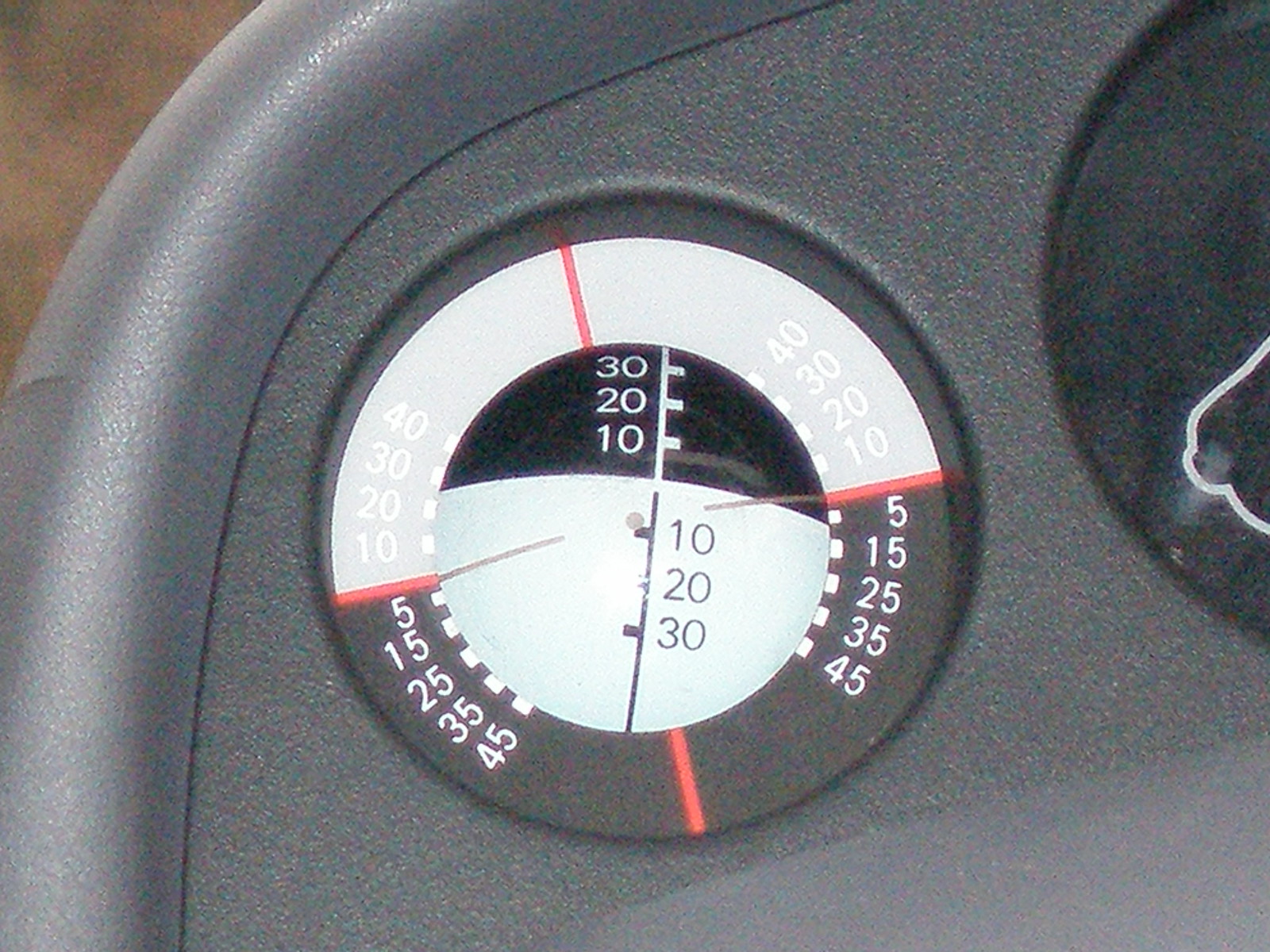This image captures a round gauge set in an indoor environment. The gauge's outer edge features a top portion outlined in light gray and a bottom portion in dark gray. The light gray upper section displays the numbers 10, 20, and 30 prominently, while the dark gray lower section features the numbers 10, 20, and 30 as well. Surrounding the outer ring, on both the left and right, the numbers 40, 30, 20, and 10 are visible on the light gray upper portion, whereas 5, 15, 25, 35, and 45 are shown on the dark gray lower portion. Four red lines accentuate each quadrant of the circular gauge, enhancing the visual guide. The background of the gauge consists of varying shades of gray, contributing to the detailed and intricate design.